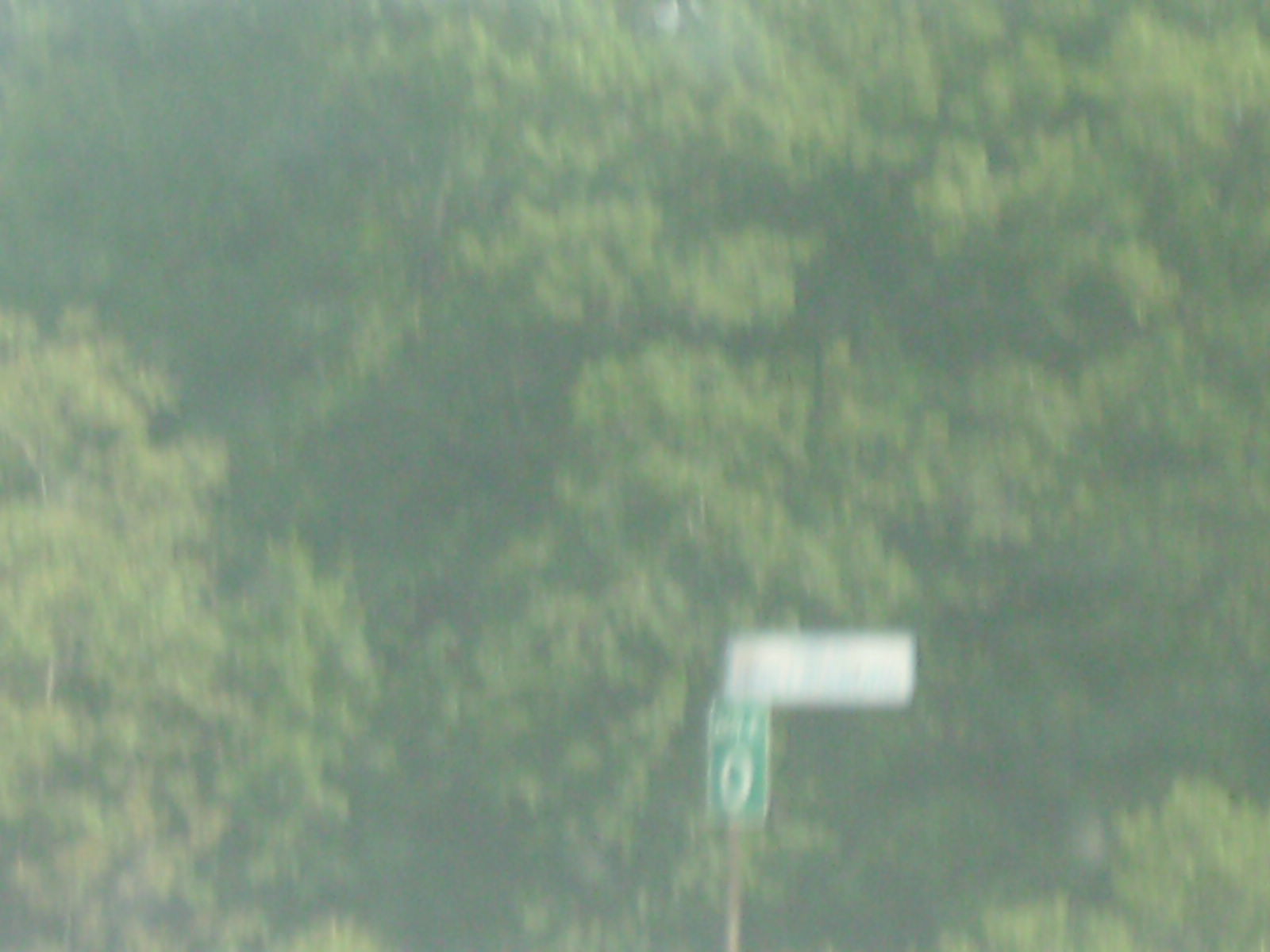A blurry daytime photograph depicts a lush forest background with various shades of green, ranging from light to dark. In the foreground, there is a sign at the bottom featuring the number "0" in green against a white background. Interspersed through the image are patches of white and black, possibly due to lighting or camera artifacts.